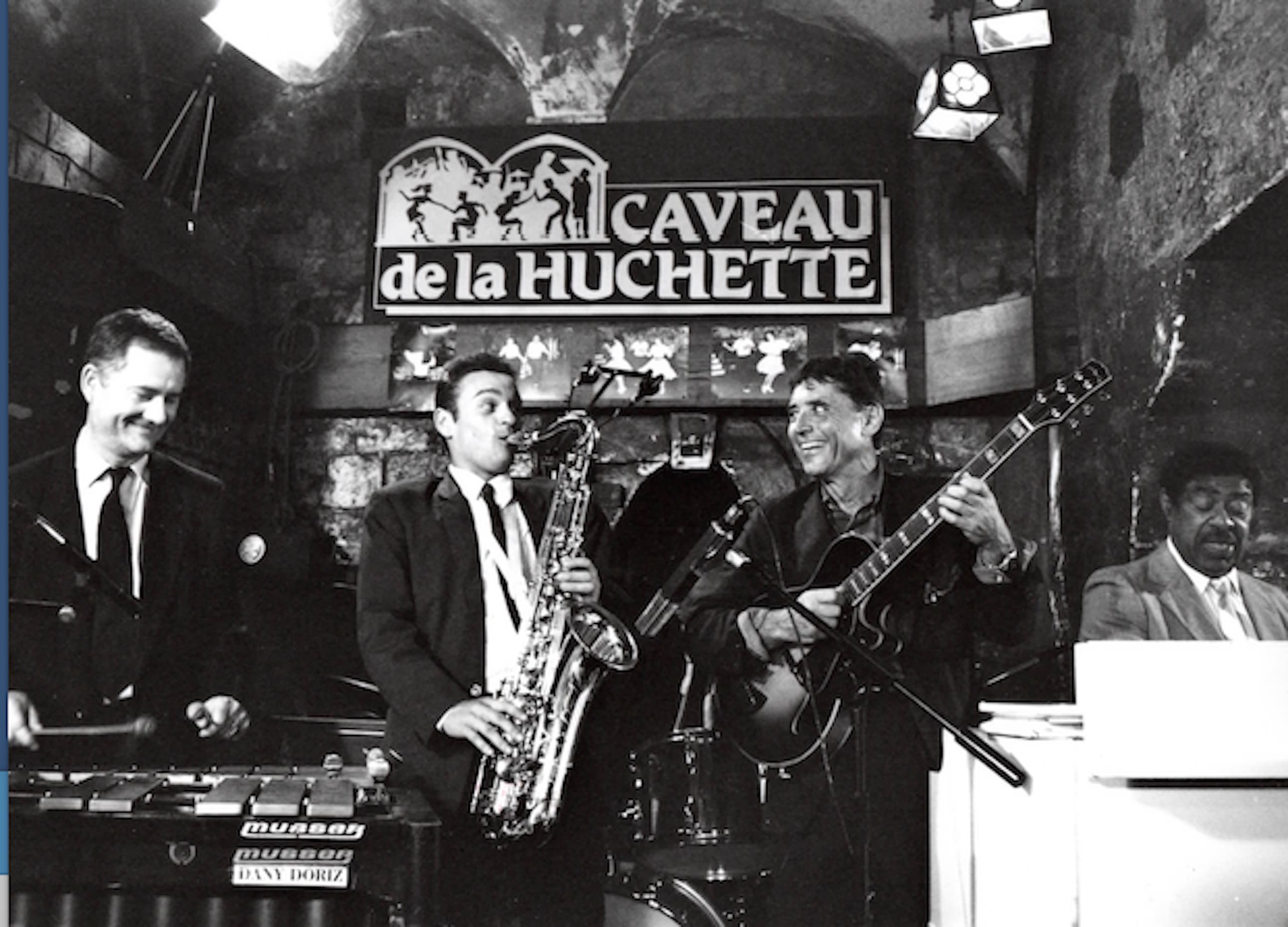In this striking black and white photograph, a live music band delivers a captivating performance in what appears to be an old castle-like interior with gray walls. All the band members are dressed in modern, contemporary suits and ties. Positioned from left to right, the first musician appears to be playing an instrument with a pong-like drumstick, possibly a xylophone. Next to him stands a white, Caucasian man intensely playing a trumpet or trombone. Moving further to the right is another Caucasian man with dark hair, expertly strumming a guitar, a microphone prominently jutting out in front of him. Finally, seated behind the piano and facing the audience is an African American pianist, adding depth and emotion to the musical experience. Hanging above them, a black and white sign reads "CAVEAU DE LA HUCHETTE," embedding a sense of place and history into the vibrant scene.